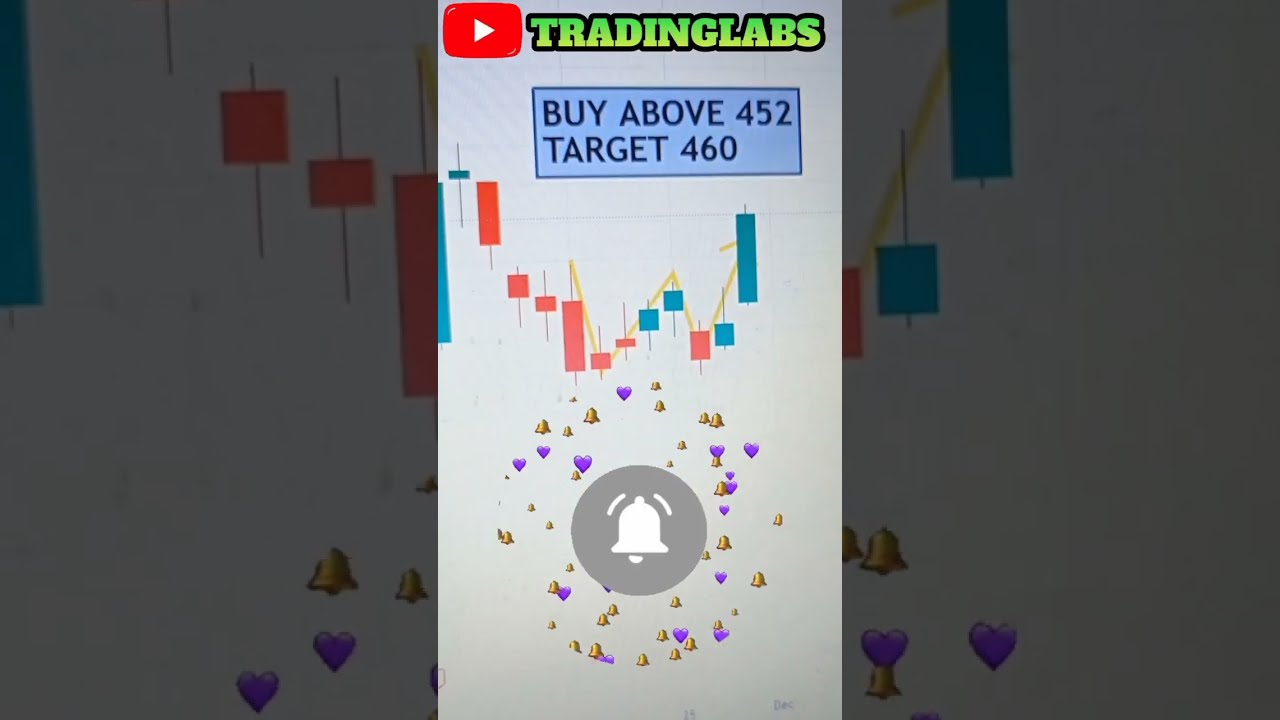The image resembles a video interface framed in a blue rectangular area with various sections depicting trading information and decorative elements. In the top left corner of the central area, there's a red rectangle with a white play arrow, signifying a video playback feature. Next to it, "Trading Labs" is written in bright neon green. Just below that, a box displays the text "Buy Above $4.52" and "Target $460."

Below this text box, there is a bar chart featuring a sequence of colored bars. Starting from the left, there is a very long blue bar, followed by an alternating pattern of shorter blue and red bars. Near the right side, another long blue bar is visible, indicating significant trading activity.

At the bottom of the image, there is a gray circle containing a white bell icon. The bell is flanked on both sides by white lines, designed to represent ringing or movement. Surrounding the bell are numerous tiny floating gold bells and purple hearts, ranging in size from very small to even smaller. These elements collectively create a festive atmosphere, reminiscent of party decorations.

The left and right thirds of the image appear to be enlargements of the central third, giving a blown-up, zoomed-in effect to the picture's content.